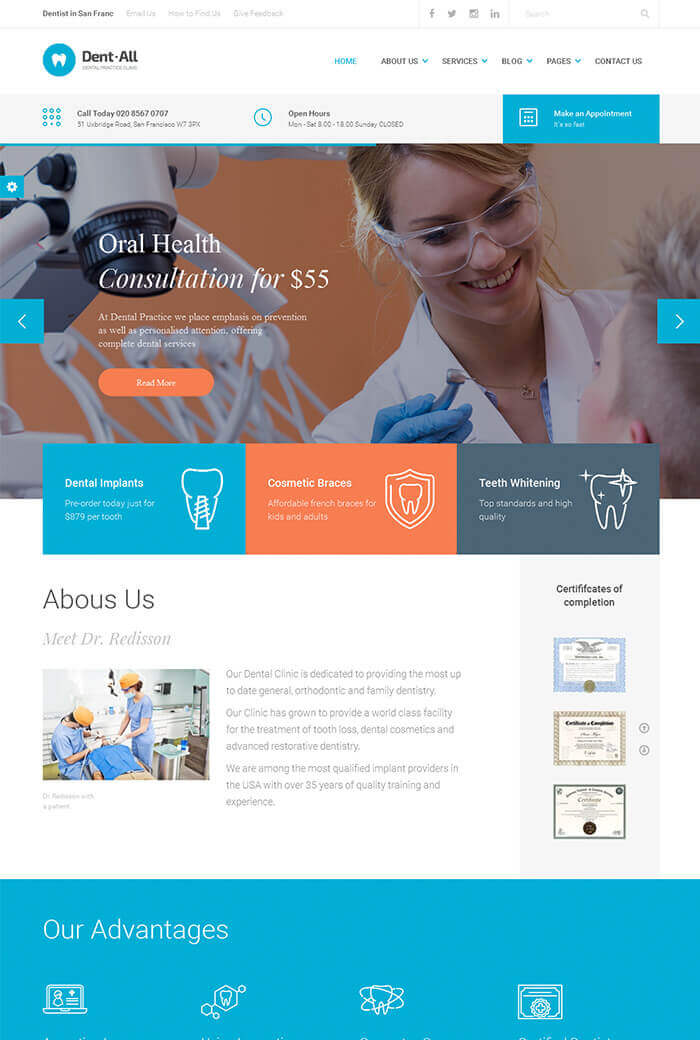---

**Website of Dental Dentists in San Francisco**

- **Contact Information:**   
  - **Email Us:** [Email link]
  - **Phone:** 020-8567-0707
  - **Address:** 51 Old Bridge Road, San Francisco, CA

- **Hours of Operation:**   
  - **Monday to Saturday:** 8:00 AM - 6:00 PM
  - **Sunday:** Closed

- **Navigation Links:**  
  - **Home**
  - **About Us**
  - **Services**
  - **Blog**
  - **Contact Us**
  - **Give Feedback**
  - **How to Find Us**

- **Call to Action:**  
  - **Call Today:** 020-8567-0707

**About Our Clinic:**

Our dental practice is devoted to offering a comprehensive range of services with a strong emphasis on prevention and personalized care. We provide an array of complete dental services including general dentistry, orthodontics, and family dentistry. Our clinic has grown into a world-class facility specializing in the treatment of tooth loss, dental cosmetics, and advanced restorative dentistry.

**Meet Dr. Reddison:**

- **Dr. Reddison** is a leading figure in our dental practice, dedicated to providing the latest in dental care and maintaining a high standard of patient-focused treatment.

**Special Features:**

- We offer oral health consultations conducted by experienced fibrologists, with a focus on preventive care and individualized attention.
- Our clinic is equipped with state-of-the-art technology to ensure the best possible outcomes in dental wellbeing.

**Providing Advanced Dental Solutions:**

Our mission is to bring cutting-edge dental care to the community, ensuring that every patient receives the best possible treatment in a comfortable and welcoming environment.

---

This caption is intended to give a comprehensive overview of the website's offerings, services, contact details, and the core values of the dental practice.